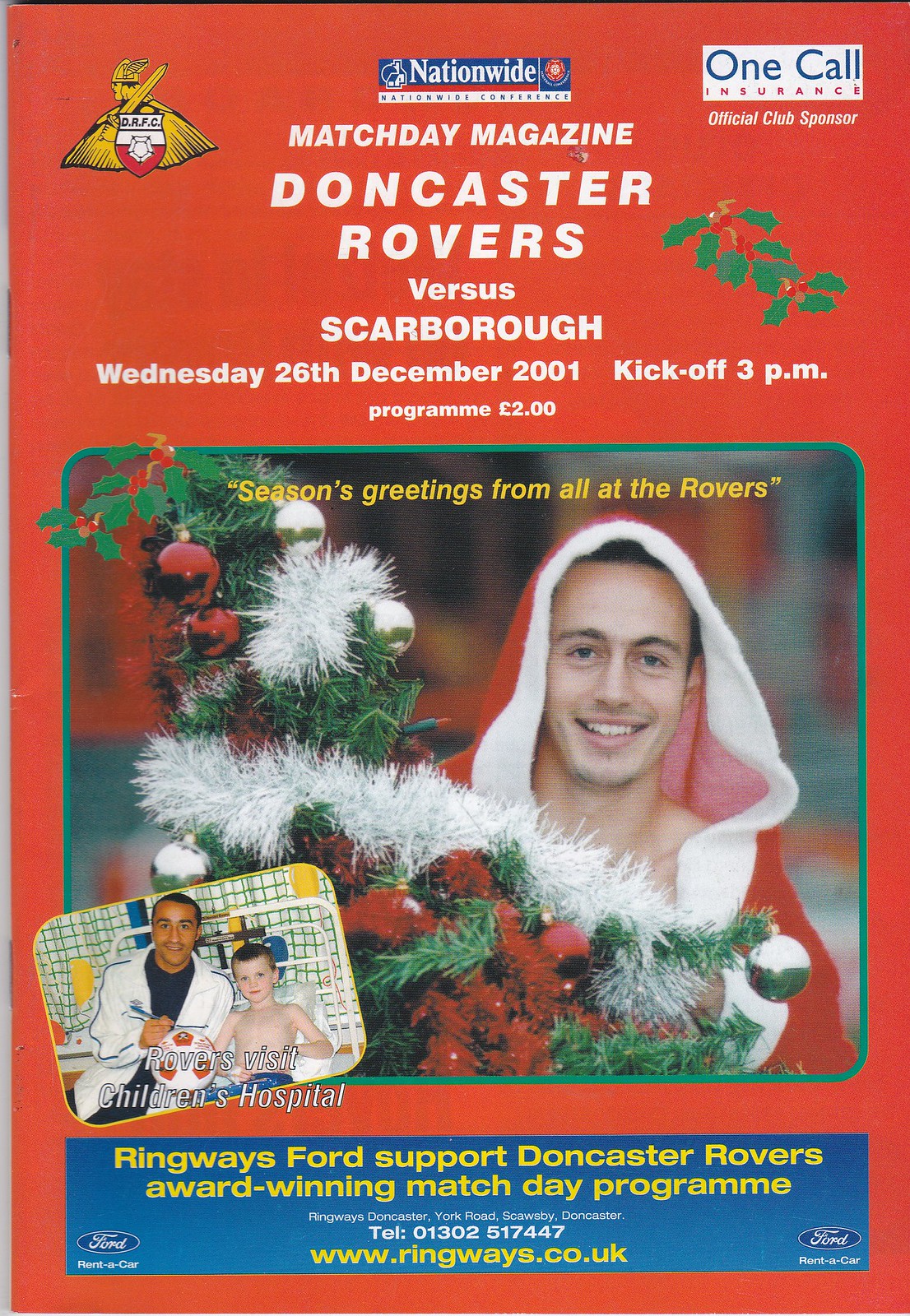The image depicts the cover of a Matchday Magazine for a soccer game featuring the Doncaster Rovers versus Scarborough, with a prominently orange background emblazoned with logos and advertisements. At the top, a blue banner displays "Nationwide," followed by a white rectangle reading "OneCall Insurance, official club sponsor." In white text down the center, it announces "Matchday Magazine: Doncaster Rovers vs. Scarborough, Wednesday, 26 December, 2001, kickoff 3 p.m., program two pounds."

Dominating the center is a festive square photograph of a man clad in a Santa-style red and white bathrobe, hood pulled up over his head akin to a boxer, bearing a smile with a decorated Christmas tree adorned with white and red garlands, baubles, and tinsel behind him. Above this image, yellow text wishes "Season's Greetings from all of the Rovers."

A smaller inset photo in the bottom left depicts a player visiting the children’s hospital, interacting with a young patient, underlined by the text "Rovers Visit Children's Hospital." Further down, a blue banner with yellow text advertises "Ringways Ford support Doncaster Rovers award-winning matchday program," providing contact details and the website www.ringways.co.uk. Two Ford logos signifying "Ford Rent-A-Car" visually balance the bottom corners of the cover. This comprehensive composition captures the festive spirit, community involvement, and critical match information for fans and attendees.